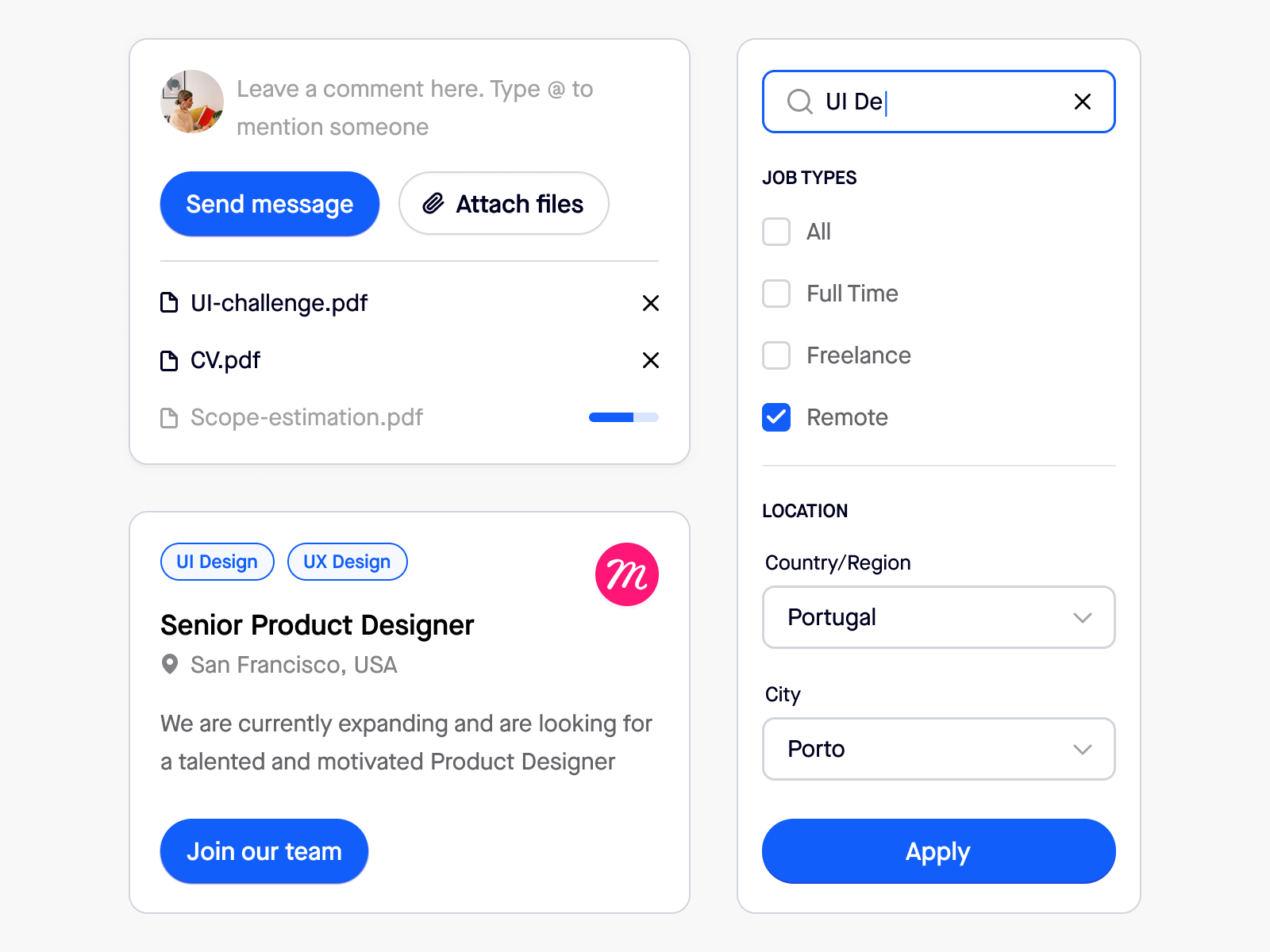This is a detailed caption for an image profiling a person offering a service:

---

The profile interface of a service provider is carefully organized into three sections. At the top section on the left, there are two boxes. The first box features the provider's profile photo accompanied by a prompt that says, "Leave a comment here. Type @ to mention someone." Below this, there is a blue "Send Message" button, and to its right, there is a white "Attach Files" button with a paperclip icon. A thin light gray line separates this area from a list of document icons underneath it. The documents listed include "UI-challenge.pdf," "cv.pdf," and "scope-estimation.pdf," each having a closeout cross to the right. A status bar indicates that the last document is currently loading and is a little more than halfway done.

Below this, the second box starts with two buttons labeled "UI Design" and "UX Design," followed by the title "Senior Product Designer." A location icon is also present with the text "San Francisco, USA." To the right, there's a pink circle with an elaborate "M" inside. Below this is a recruitment message that reads, "We are currently expanding and are looking for a talented and motivated product designer," accompanied by a "Join Our Team" button.

The right section prominently features a search bar with the text "UI DE," where the cursor is currently active. Below this, categories for job types are listed vertically with checkboxes: "All," "Full-time," "Freelance," and "Remote," with the "Remote" option checked. Another thin gray line separates this from the next category, which includes "Location." Two drop-down menus are available for location selection: one for "Country/Region" showing "Portugal" and another for "City," showing "Porto." An "Apply" button is positioned at the bottom.

---